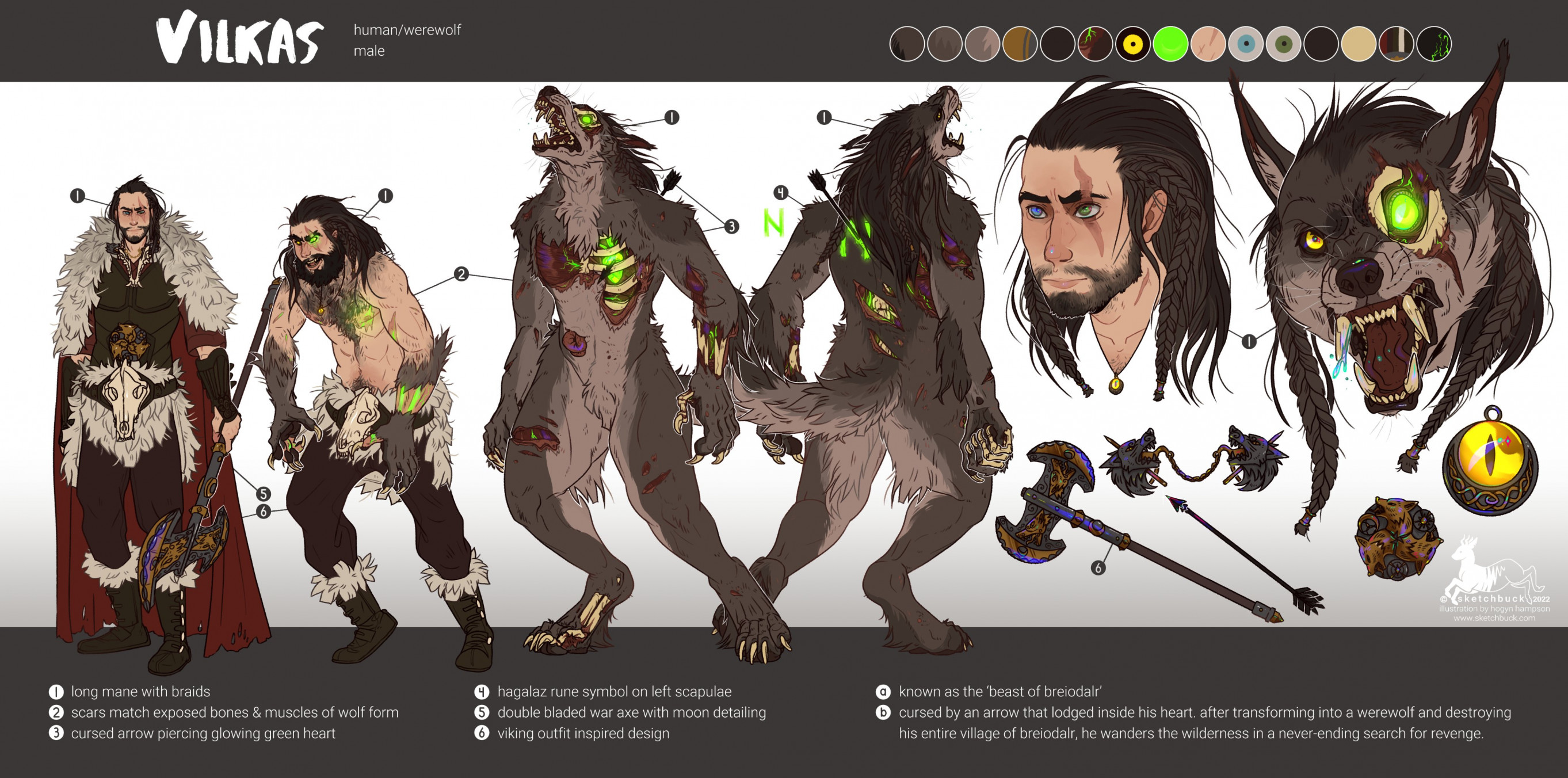This image appears to be a dramatic, realistic, fantasy cartoon character sheet for Vilkas, a male human-werewolf hybrid. At the top, the text "Vilkas, Human/Werewolf, Male" is prominently displayed. The sequence of detailed illustrations showcases Vilkas's transformation from human to werewolf, starting with his human form on the left, progressing through various stages of the transformation, and culminating in a depiction of both the human and werewolf heads on the far right. The color palette consists mainly of grays and browns, complementing the character's hair and fur tones. 

Various weapons and tools are illustrated around the character, including a battle axe and a cursed arrow piercing a glowing green heart. Detailed descriptions accompany each illustration, with lines linking numbered points on the character to corresponding notes below. These notes include phrases like "long mane with braids," "scars match exposed bones and muscle of wolf form," and "cursed arrow piercing." Additional text describes elements such as Viking outfits and other symbols, contributing to the backstory and characteristics of Vilkas.